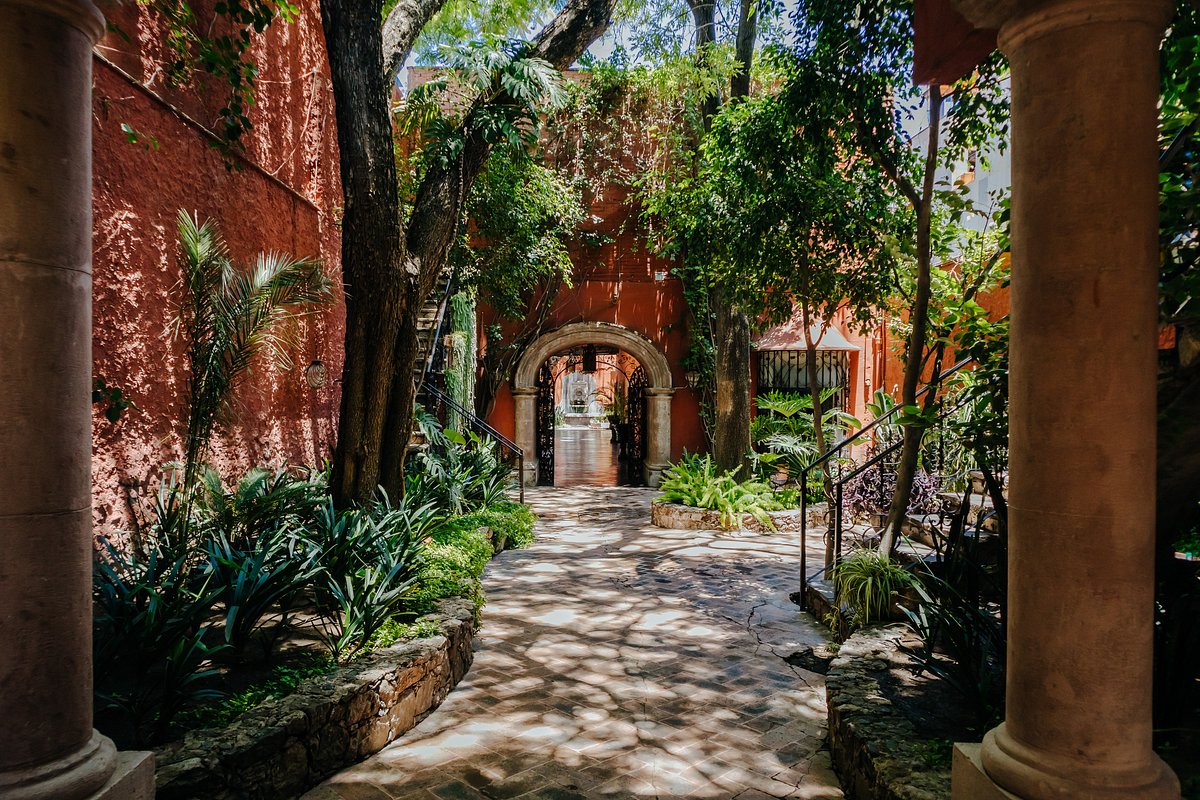The image captures a warm, Spanish-style courtyard, perhaps part of a villa, hotel, or resort, characterized by its red clay stucco structures and vibrant greenery. Dominating the scene is a long, gray stone-tiled walkway, patterned in a herringbone design, bisected by shadows from the surrounding trees. The walkway, rising slightly before turning right into four barely visible steps, leads towards a distant brown building with a white-bordered entryway flanked by columns. This building, draped with lush greenery, features an archway and a barred window partially obscured by plant life. At the forefront, two substantial grayish-black concrete pillars frame the walkway, accompanied by lush, small green plants and a prominent tree branching overhead. On either side, additional greenery, including palm-like plants, adds to the courtyard’s rich, verdant atmosphere. The right side also features a black metal railing leading from the steps, with possible hints of flowering plants in the corners. The architecture and vegetation suggest a setting in a warm climate, with influences that might be Mexican or Spanish, under a mostly obscured blue sky.